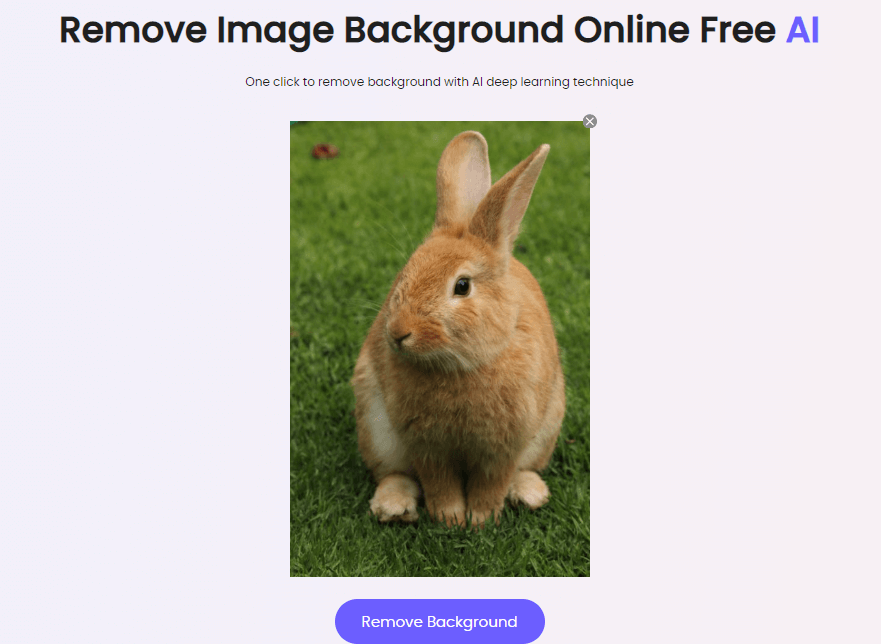A screenshot in landscape orientation showcases an image editing interface with a light pinkish-purple background. At the center, there's an image of an orange rabbit centered on vibrant green grass, facing towards the left. The rabbit, which is slightly squatting and upright, reveals one eye, its nose, four feet, and both ears. To the left of the rabbit, a red ball or flower is visible. The image of the rabbit seamlessly cuts off with no visible borders.

At the top right of the screen, there is an 'X' icon, presumably to close the interface or the image. Positioned below the rabbit's image is a prominent blue button inscribed with “Remove Background” in white text. Above the central image, black text in a simple font reads “Remove Image Background Online Free,” with the word “AI” highlighted in blue. Beneath this, in smaller black text, it states, "One click to remove background with AI deep learning techniques." This detailed visual composition centers around the rabbit, drawing attention to its surroundings and the interface elements designed for background removal using AI.